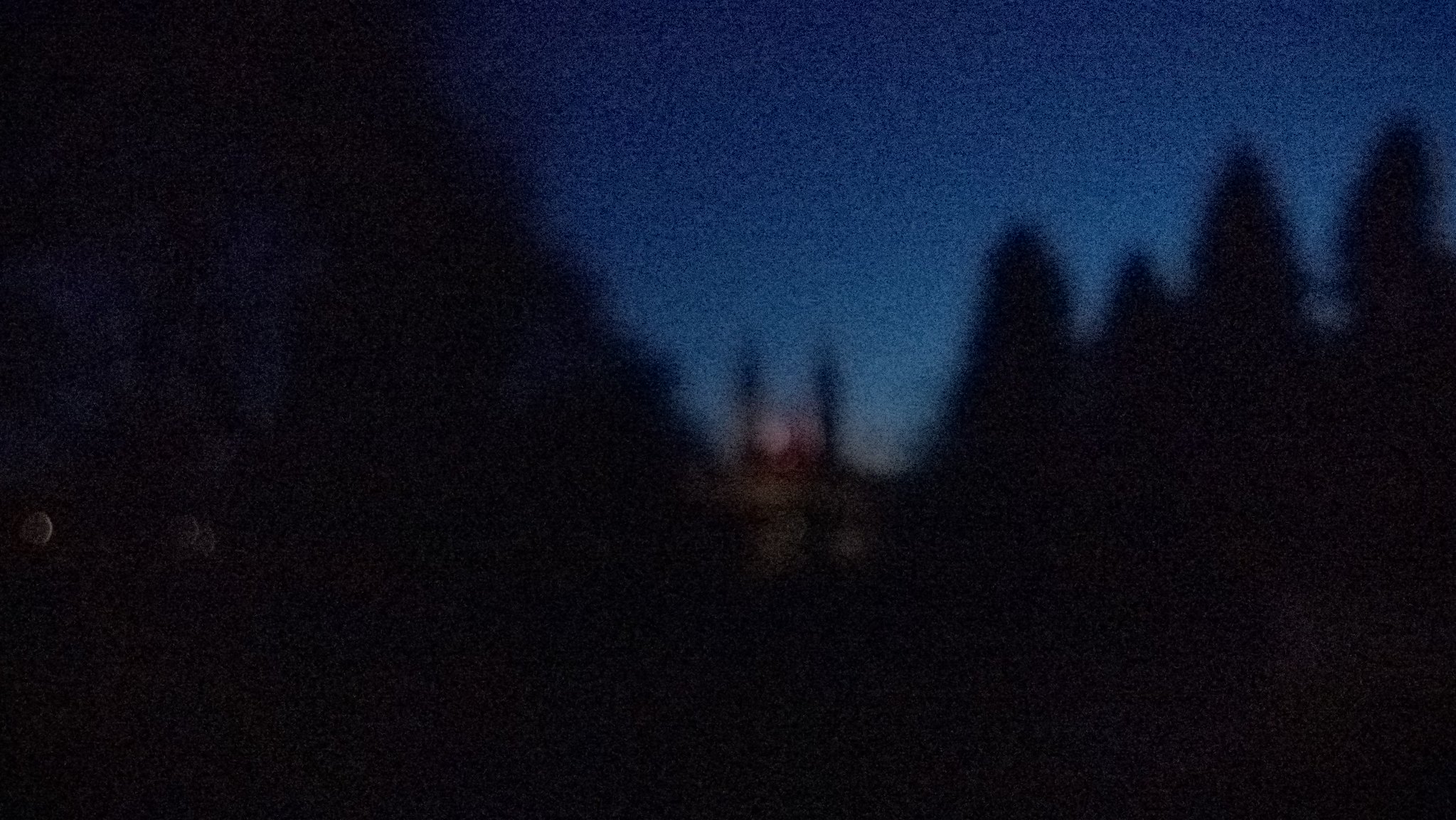A blurred nighttime photograph featuring indistinct trees flanking both sides. The trees, identifiable by their pointed tops and bulky middles, stand in contrast to the deep blue sky dotted with stars. In the center background, a structure with pointed projections is visible, creating an ambiguous silhouette against the starry night. The structure appears to be either a building or a train moving along a track, though the blurred quality leaves its exact nature open to interpretation.